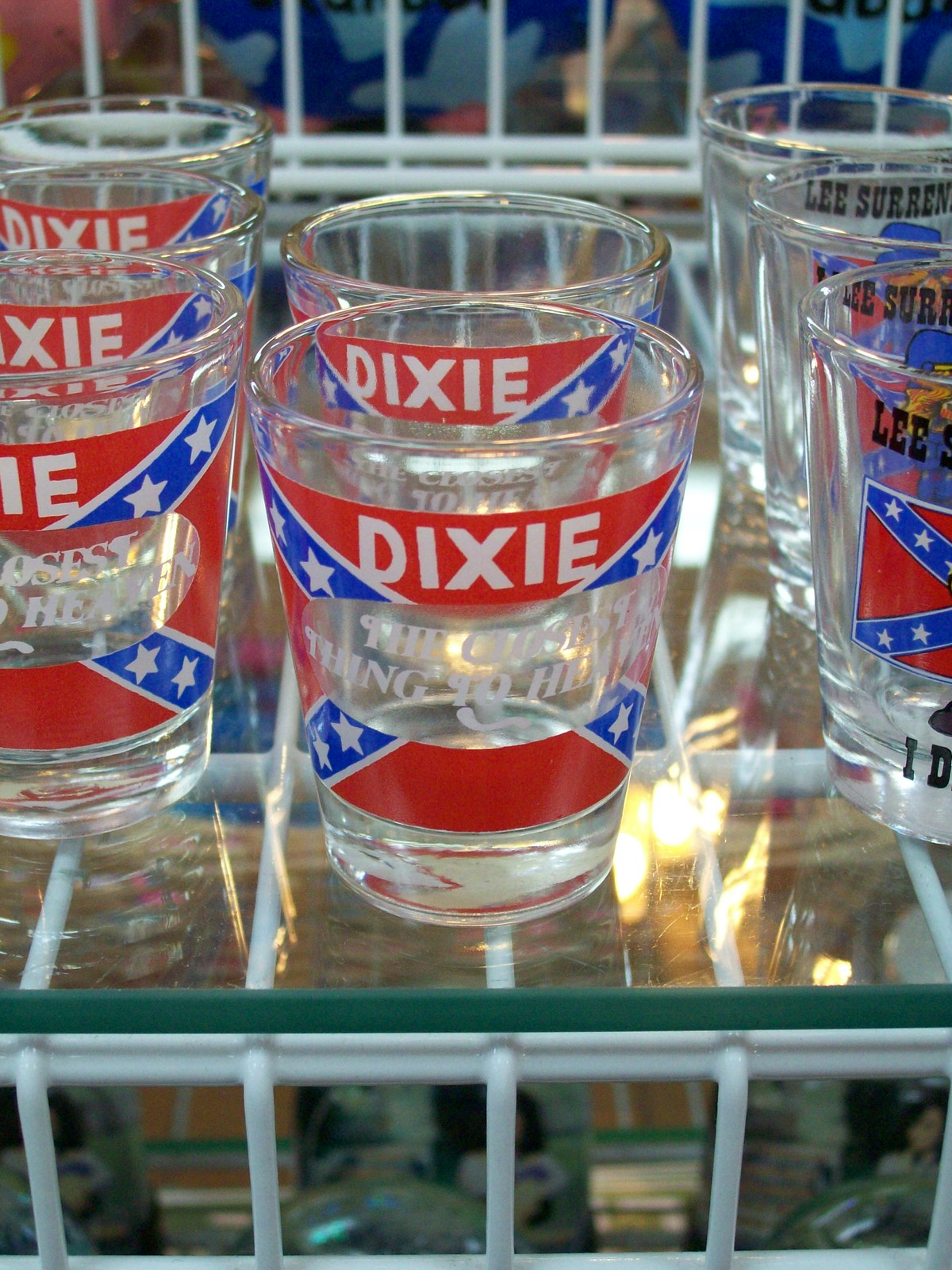This image shows a collection of shot glasses displayed on a glass-topped, white wire shelving unit, likely taken in a store setting. There are eight shot glasses in total, arranged in vertical rows with three on the left, three on the right, and two in the middle. The shot glasses on the left prominently feature a large Confederate flag with the text "Dixie" in white letters at the top. In the center of the flag, there's a cut-out text that reads "the closest thing to heaven" in a slightly fancy font. These designs are repeated across five glasses. On the right-hand side, which features the remaining three shot glasses, a Confederate flag is also visible along with partial text that reads "Lee surrenders" at the top. Another design element includes a figure dressed in a Confederate uniform, and the text "I did not" is likely present but cut off in the image. Below the shelf, there are various blurred knickknacks that are not clearly identifiable. The overall American theme, with an emphasis on Confederate imagery, is clear in the shot glass designs.